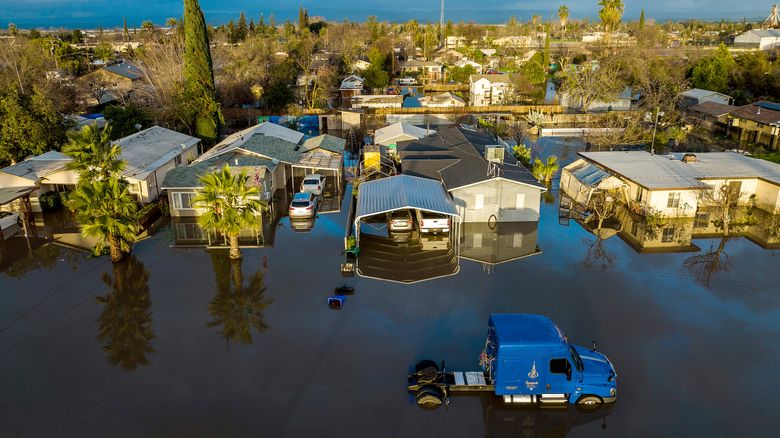This image captures a devastating flood in a small coastal town, likely in California judging by the plant life and building styles. Shot from an aerial perspective, the photograph shows an expanse of bright blue ocean at the top, contrasting sharply with the flooded neighborhood below. The floodwater, a dark bluish-black, has submerged the streets and reflects the surrounding buildings and trees, giving the impression that the town has been engulfed by the sea. The area predominantly features small single-family homes or mobile homes, some bordered by wooden fences and surrounded by trees, including visible palm trees which suggest a tropical setting. A blue semi-truck, without a trailer and partially submerged up to its tires, can be seen near the bottom center of the image. The water level appears substantial, reaching several feet deep in some areas; it laps halfway up the wheels of vehicles and floods through carports. This scene reflects a moment of severe flooding, illustrating the vulnerability of this picturesque yet inundated coastal town.